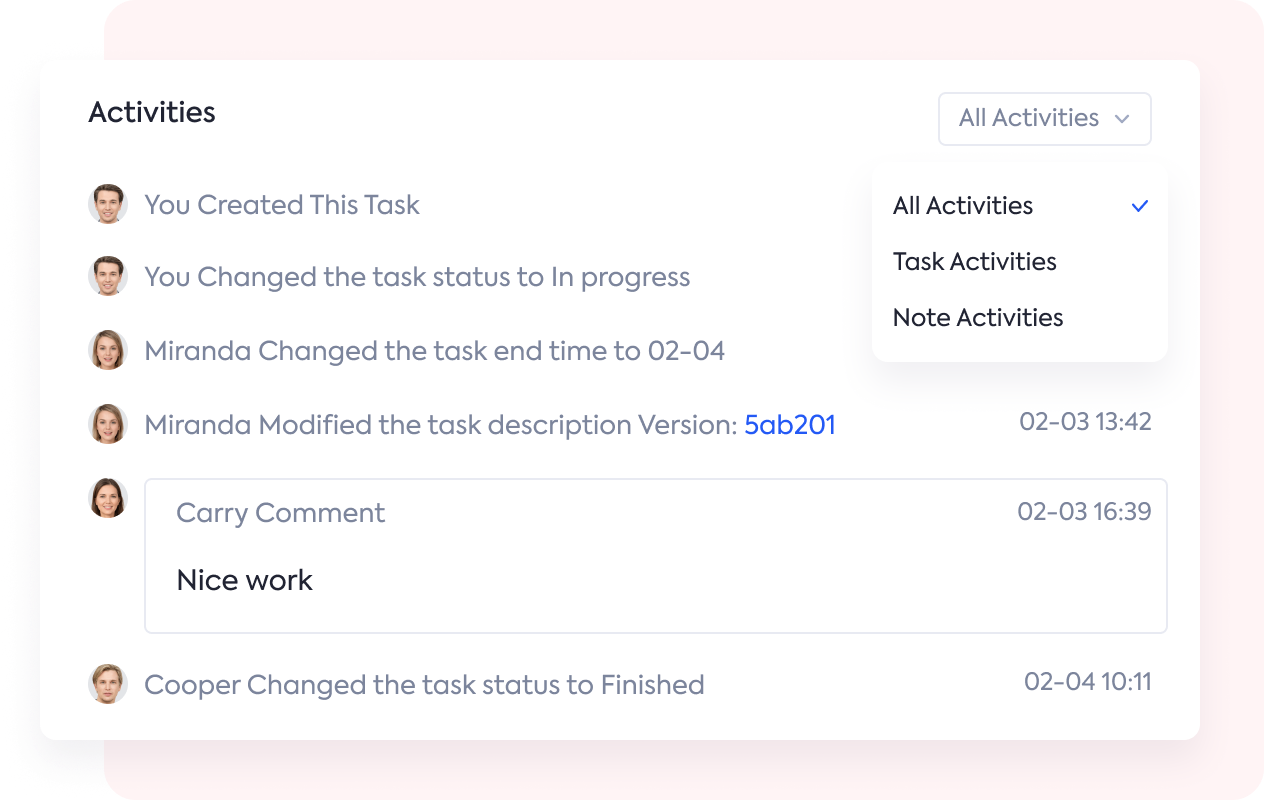The background of the box is a light pink color. On the left side, there's a white box with the word "Activities" written in black text. Below this, there's an image of a man's face inside a small circle, accompanied by the text "You created this task." 

Immediately following, there's another instance of the man's image with the text "You changed the task status to 'In Progress.'" 

Next, there's an image of a woman's face inside a small circle. She has brown hair and a neutral expression on her face. Beside this image, the text reads "Miranda changed the task end time to 02-04." Further down, Miranda's name appears again, this time indicating she "modified the task description version," with the version number "5AB201" highlighted in blue. 

To the right of this information, the date "02-03" and time "13:42" are displayed. Below this, another image of the same woman’s face appears inside a circle, with the text "Carry commented" below it. In darker black text, it reads "Nice work." To the right, the date "02-03" and time "16:39" are shown. 

Lastly, there's an image of a man with brown hair and a neutral expression. The text next to his image reads "Cooper changed the task status to 'Finished.'" This marks the end of the activity log.